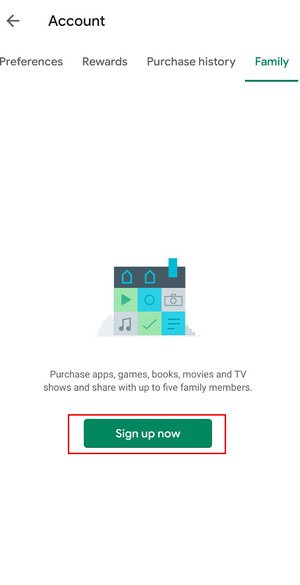The image is a screenshot of a webpage captured on a smartphone, showcasing a primarily white interface that is  rectangular in shape. At the top of the page, there is a navigation bar with gray text options labeled 'Preferences,' 'Rewards,' 'Purchase History,' and 'Family.' The 'Family' option stands out as it is highlighted in green and underlined. 

Towards the bottom of the page, there is a prominent red-outlined banner that includes a green button with the text 'Sign Up Now' in white lettering. The banner provides information, stating: "Purchase Apps, Games, Books, Movies, and TV Shows and share with up to five members."

Superimposed on the page are several squared boxes, each containing distinct symbols. One box features a vertical turquoise rectangle resembling a house. Two other boxes display blue, house-shaped icons. Additionally, there are boxes with varied symbols including a green arrow, a green check mark, and a blue circle.